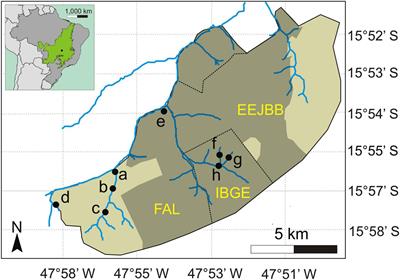This image features a detailed map with various geographic and cartographic elements. Centrally displayed is a rectangular map that is a close-up of a region within a larger continent, likely Brazil, as indicated by the shaded area in the upper left corner. The map includes a scale in the lower right-hand corner, denoted by a five-kilometer bar divided into white and black segments. Longitude markings such as 47°58'W, 55°W, 53°W, and 51°W, as well as latitude ranges from 15°52'S to 15°58'S, are indicated along the borders. A compass with an arrow pointing north is located in the lower left-hand corner.

There are numerous features within the map, such as a network of blue lines representing rivers and several black dots labeled with letters from A to H across a landmass. Additionally, the map contains acronyms including F-A-L, I-B-G-E, and E-E-J-B-B. A prominently green-shaded, kidney-shaped region is mapped out, lying on a background gridded with latitude and longitude lines. Specific areas are emphasized in yellow capital letters, providing a clear, intricate depiction of the region.